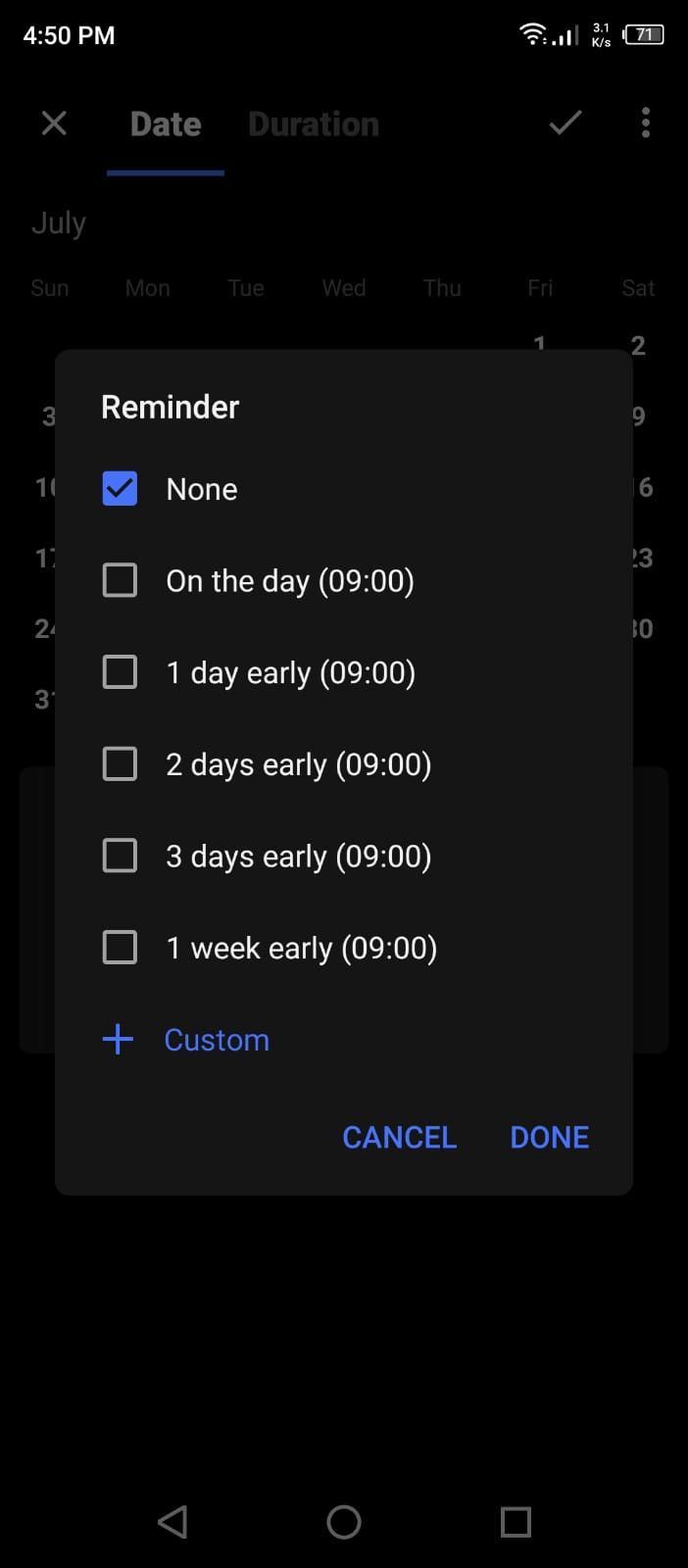A screenshot of a cell phone displays various interface elements. In the upper left-hand corner, the current time is visible: 4:50 p.m. On the upper right-hand corner, there is a series of status icons, including a Wi-Fi logo, a cell phone reception icon, and a battery icon. Just beneath these icons, there is a small icon that shows "3.1 K/S." Directly below the time display on the left, an "X" close icon is present.

There is a date and duration tab below the top bar, where the date tab is currently selected and highlighted in white font with a blue underline. Adjacent to the battery icon on the right is a checkbox followed by a vertical three-dot menu, indicating additional options.

At the center of the screen, a pop-up menu is displayed titled "Reminder." This menu offers various options to set reminders: "None," "On the day," "One day early," "Two days early," "Three days early," and "One week early." At the bottom of this pop-up menu, buttons labeled "Cancel," "Done," and "Custom" are available for further actions. The overall layout provides a clear, organized view of the phone's interface and reminder settings.